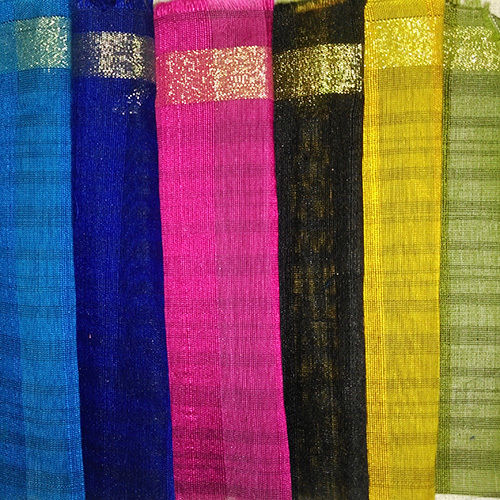The image displays an ornate arrangement of six different fabrics, likely intended for drapes or curtains. From left to right, the colors are light blue, dark blue, pink, black, yellow, and green. Each fabric features horizontal stripes with alternating shades, creating a two-tone effect. A shiny gold strip runs along the top edge of all the fabrics, adding a touch of elegance. The fabrics have a sheer, silky texture, allowing them to be slightly transparent and enabling layers of colors to intermingle. Additionally, glitter embellishes the blue fabrics, cascading from top to bottom, enhancing the luxurious feel of the presentation.